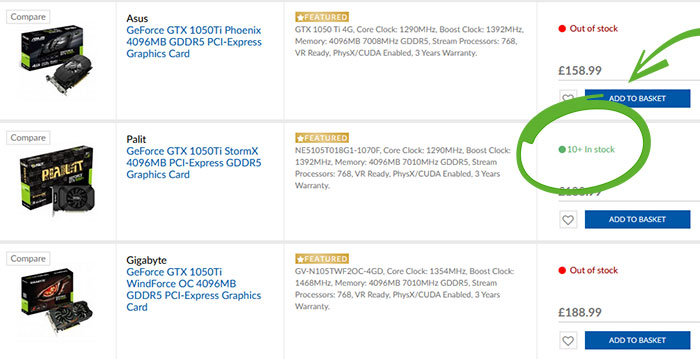In the screenshot, three different graphics card products are being compared. The first product is identified as a GeForce GTX 1050 Phoenix Express graphics card, priced at £158. However, this item is marked as "Out of Stock" with a gold box featuring a white star labeled "Featured." Next to the price, there is a blue "Add to Cart" button accompanied by a heart icon for saving the item to a favorites list. The final product in the lineup is a Gigabyte graphics card, which is also out of stock.

Between these two, the second product differs, clearly highlighted with a green circle and an arrow pointing to the text "10 in stock." This middle item is more affordable compared to the others. Although the brands of the middle and the last products are not specified, the visual cues make it clear that the middle graphics card is currently available for purchase.